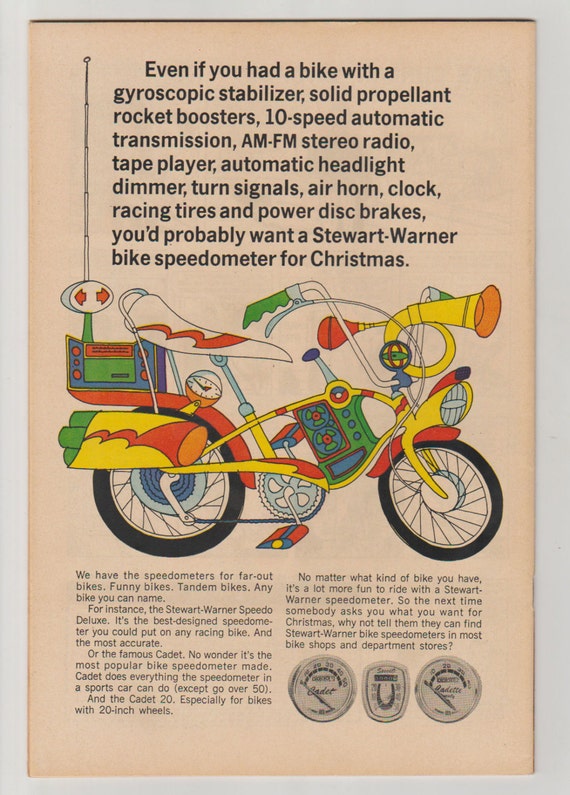This image from an old, yellowed magazine, likely from the 1960s, features an advertisement for a Stuart Warner bike speedometer. The rectangular image, measuring about six inches high by four inches wide, is framed by a thin light gray border. At the top, bold black text reads: "Even if you had a bike with a gyroscopic stabilizer, solid propellant rocket boosters, 10-speed automatic transmission, AM/FM stereo radio, tape player, automatic headlight dimmer, turn signals, air horn, clock, racing tires, and power disc brakes, you'd probably want a Stuart Warner bike speedometer for Christmas." Below this text is a vibrant, hand-drawn, cartoon-like image of a highly accessorized bike. The bike boasts a yellow body, long white handlebars ending in green grips, a banana seat, an antenna at the back, black tires, orange pedals and brakes, a white metallic gear, and a dark gray chain. The bike also features colorful elements such as a multi-hued radio mounted on the back. Underneath the illustration, two additional columns of text describe the speedometers. In the lower right corner, three black and white speedometers labeled "Cadet" are displayed.